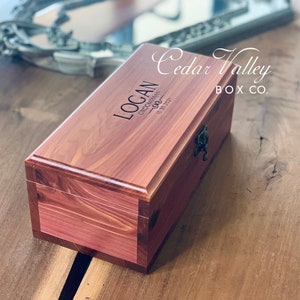The image is an advertising photograph featuring a polished, reddish-toned cedar storage box with a black latch and the name "Logan" engraved on the top. The box, suitable for holding jewelry or small trinkets, is placed on a brown wooden table that slightly contrasts in color. Superimposed on the image, above the box and table, are the words "Cedar Valley Box Co." in white cursive font. In the background, there is an intricately detailed silver tray or possibly a mirror, partially visible and lying flat on the table.